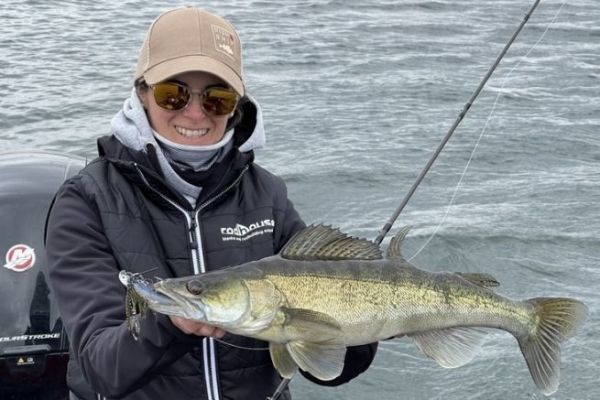A woman is photographed on a boat, proudly displaying a large fish she has caught. She wears a tan-colored baseball cap with an unreadable square logo and round, brown-tinted sunglasses. Her attire includes a black lightweight jacket with a gray hood and white writing on the chest, slightly blurred and indistinct, along with a cloth pulled up around her chin for warmth. She is smiling broadly, revealing her teeth. The fish, held horizontally in her hands, has a pointy nose, a dark gray top, speckled brown sides, and a silver underbelly, with a hook still visible in its mouth. The boat's black outboard motor, featuring a white and red logo with a large letter 'N,' is partially seen behind her, along with a fishing rod and its white line. The backdrop is a mix of gray and blue water, indicating a bright daylight setting without direct sunshine visible in the image.